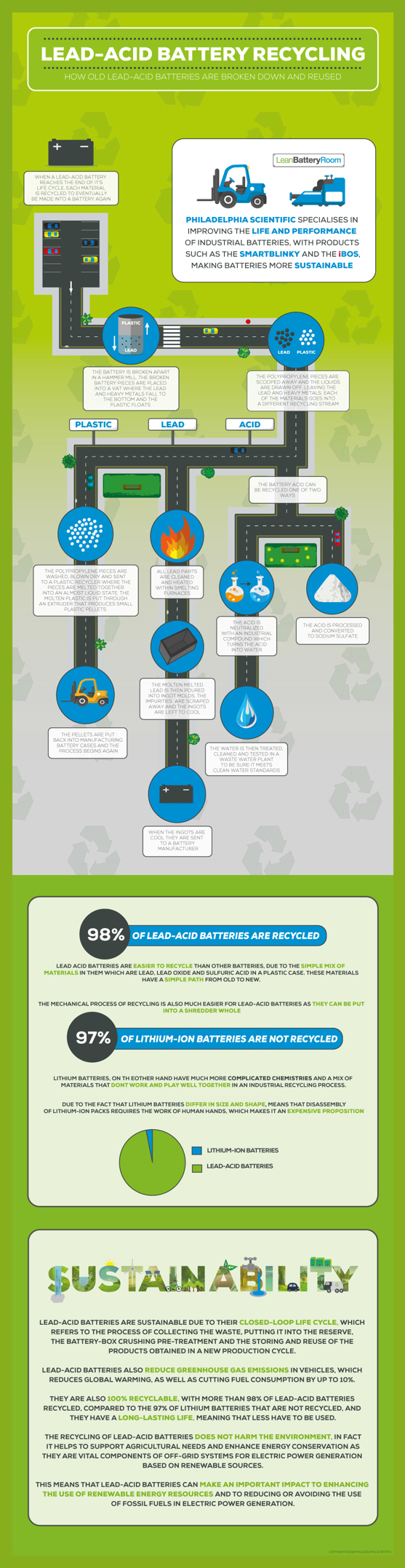The image is an advertisement flyer focused on Lead Acid Battery Recycling, presented in a vertically positioned, skinny, rectangular format with a green background. The header boldly reads "Lead Acid Battery Recycling," followed by informational text describing how lead acid batteries are broken down and reused. At the top of the flyer, there are small, unreadable lines of text beneath the header.

The main graphic in the flyer is a large informational chart divided into three sections. The largest section at the top features a gradient background shifting from green to gray, with small recycling logos subtly embedded. This section portrays a road-like diagram that illustrates the recycling stages for lead acid batteries, using a sequence of black lines and blue circles to detail the steps from collection to final processing. However, the text here is too small to decipher.

Directly below, two smaller boxes provide additional information. The first box states that 98% of lead batteries are recycled, emphasizing the efficiency in recycling these batteries. In contrast, the second box highlights a significant problem: 97% of lithium-ion batteries are not recycled. 

At the flyer’s bottom, there's a section titled "Sustainability," followed by a longer block of text in small font, which discusses Philadelphia Scientific's role in enhancing battery life and performance with products like the Smart Blinky and the iBoss, aimed at making batteries more sustainable. The details here underscore the overarching theme of the flyer, focusing on sustainable practices and efficient recycling of lead acid batteries.